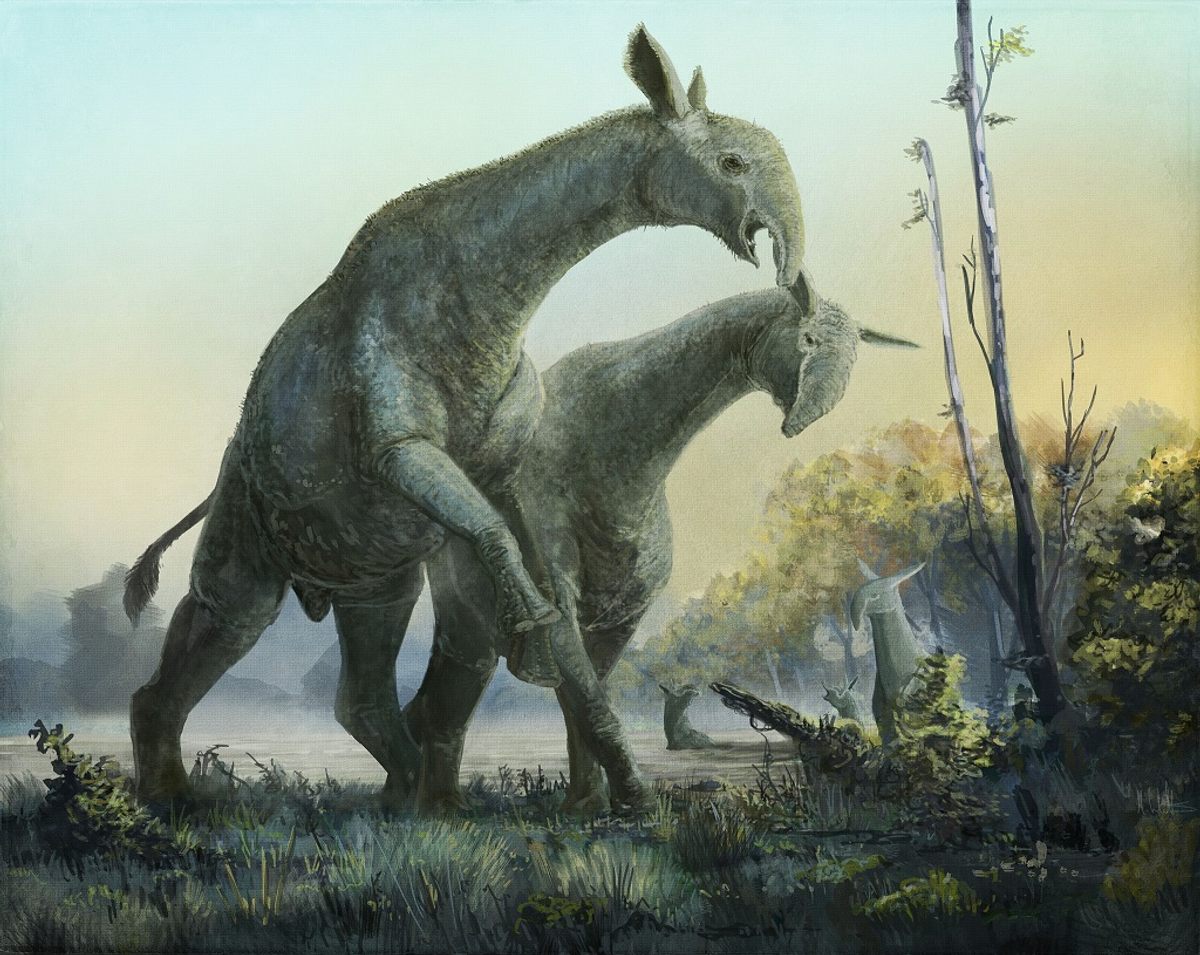The image is an artist's illustration depicting a prehistoric or fictional scene. Central to the image are two large, gray creatures reminiscent of a cross between giraffes and ant-eaters, featuring long necks, small, pretty horns, and tails similar to those of giraffes. These animals have a somewhat furry appearance on their backs, large ears, and distinctive heads with snouts resembling those of ant-eaters but shorter and more robust. They stand close together, side-by-side, with a smaller, similar creature positioned slightly to their right, suggesting a family group. The backdrop of the image showcases a misty, swamp-like environment with a hazy, bluish-yellow sky, dense with trees, and a hint of water body, enhancing the prehistoric ambiance. The scene also includes some flora, such as tall, leafless branches of a tree on the right and other grassy areas, contributing to a serene yet mysterious atmosphere.